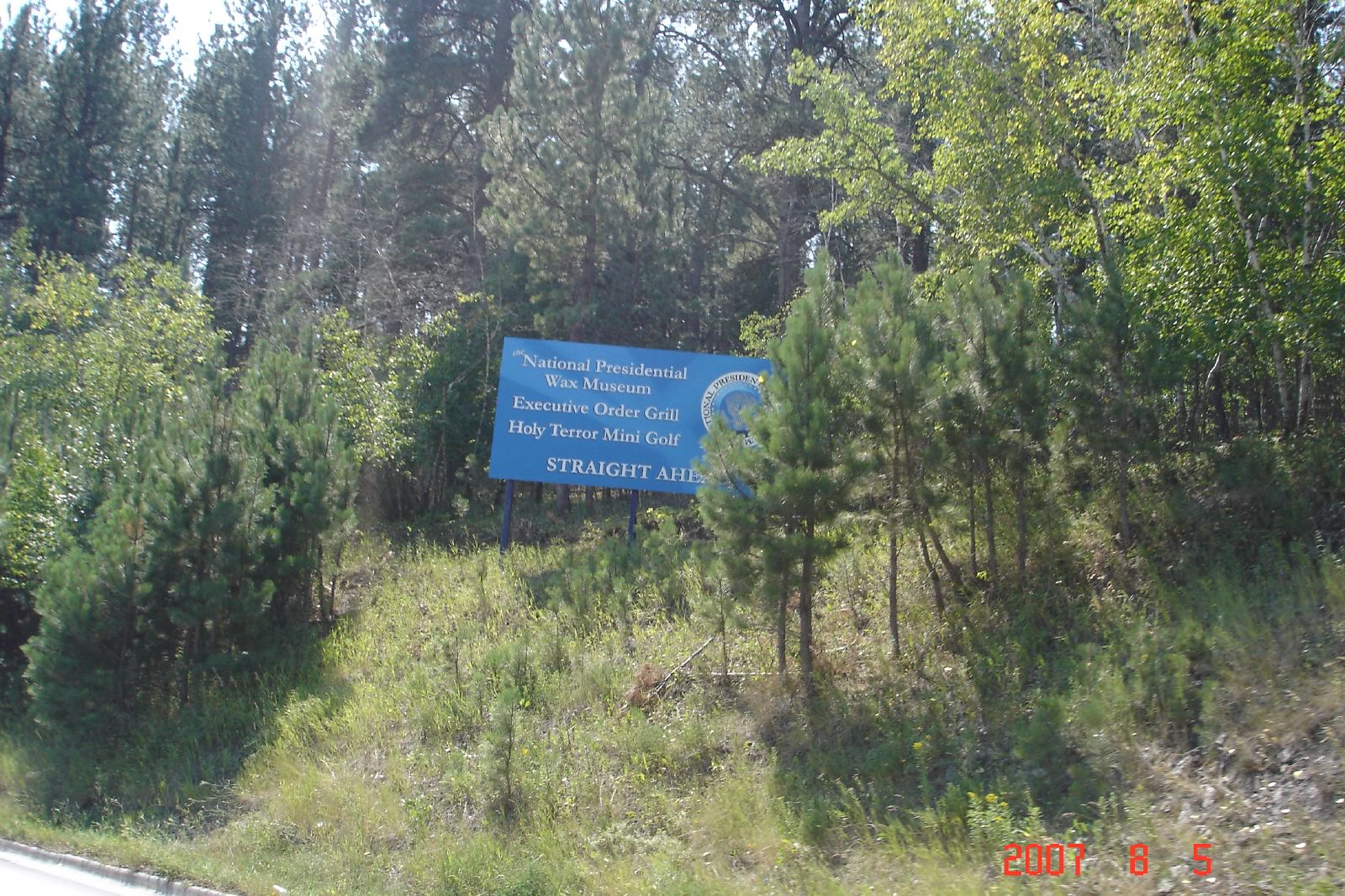A photograph captures a street scene with a billboard promoting local attractions, taken from a moving car. The motion is evident as the trees lining the street appear slightly blurred, indicating the vehicle is in motion. The billboard, predominantly blue with white text, stands against a green backdrop of leafy trees suggesting a summer day. The sign advertises the National Presidential Wax Museum, the Executive Order Grill, and the Holy Terror mini-golf, directing visitors straight ahead. The base of the image bears a red timestamp indicating the date August 5th, 2007. A curb and a gently sloping hill are visible beneath the sign, under a presumably clear blue sky.